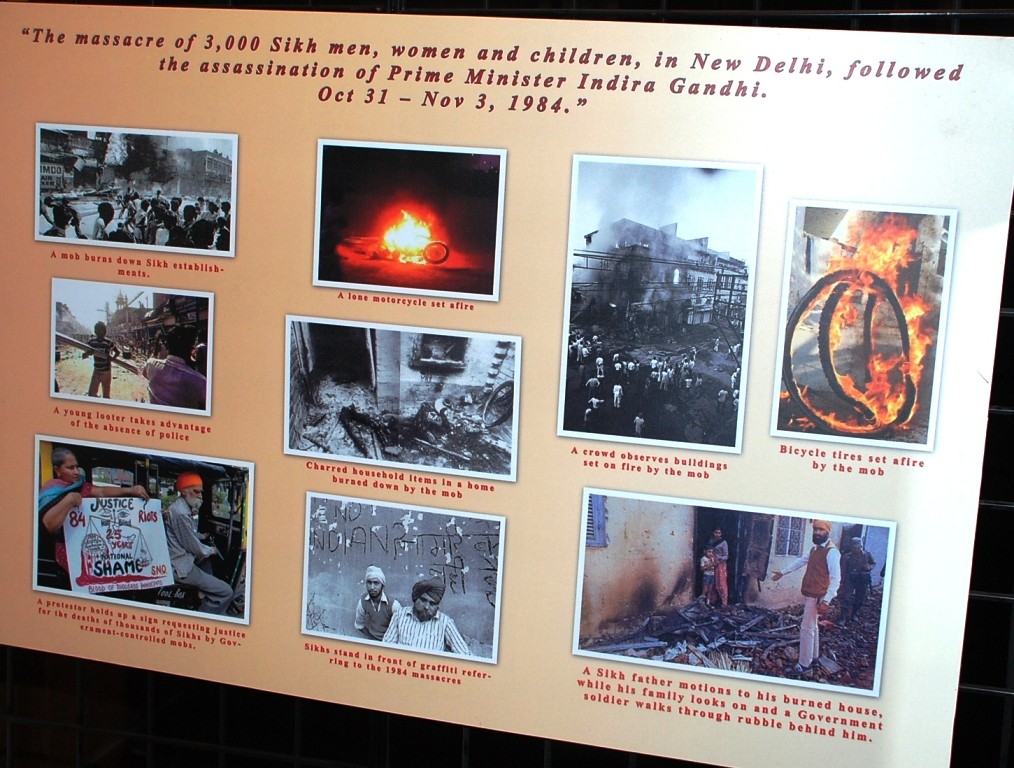This image is a detailed display featuring nine different photographs, each capturing the devastation following the massacre of 3,000 Sikh men, women, and children in New Delhi after the assassination of Prime Minister Indira Gandhi, which occurred from October 31 through November 3, 1984. At the top, in dark purple lettering, a quote highlights the tragic event: "The massacre of 3,000 Sikh men, women, and children in New Delhi followed the assassination of Prime Minister Indira Gandhi, October 31 through November 3, 1984."

The display's background is a soft peach color, set against a black backdrop. The nine photographs are a mix of black and white and color images, depicting scenes of chaos, including raging fires and smoke, and showcasing the extent of the destruction. Some of the photos' captions, though difficult to read, describe specific events captured, such as a lone motorcycle set aflame and a bicycle tire ignited by the mob, emphasizing the widespread violence and turmoil. Overall, the series of images and captions convey a harrowing and upsetting glimpse into the aftermath of this catastrophic event.